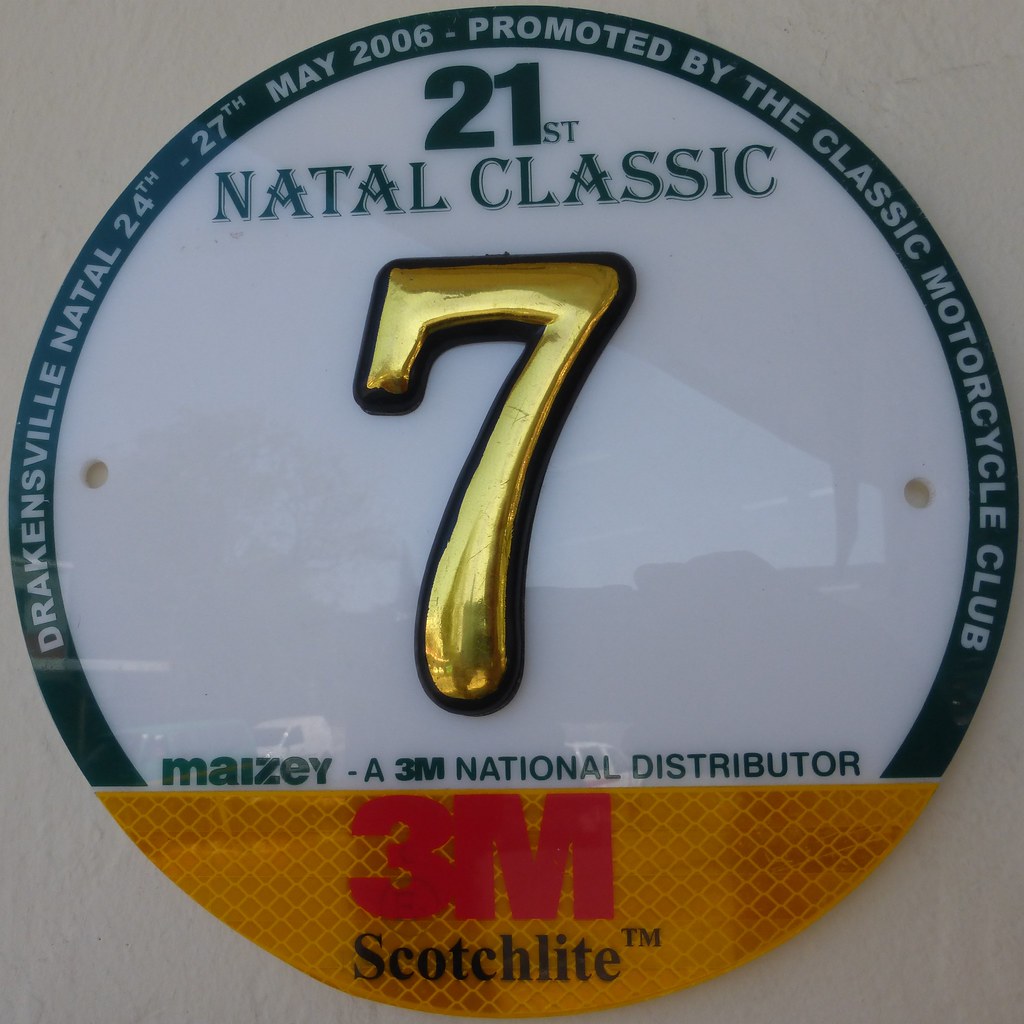The image features a circular emblem styled as a pin, commemorating the 21st Natal Classic event organized by the Classic Motorcycle Club. The emblem prominently includes a large, gold number "7" at its center. Surrounding the number, the text reads "Drakensville Noddle 24-27 May 2006 promoted by the Classic Motorcycle Club 21st Noddle Classic." At the bottom, the emblem notes "3M Scotchlite trademark" and mentions "Mazze, a 3M National Distributor," highlighting the sponsorship and possible celebration of a 7-year milestone. The design is set against a white background, which could be a wall.